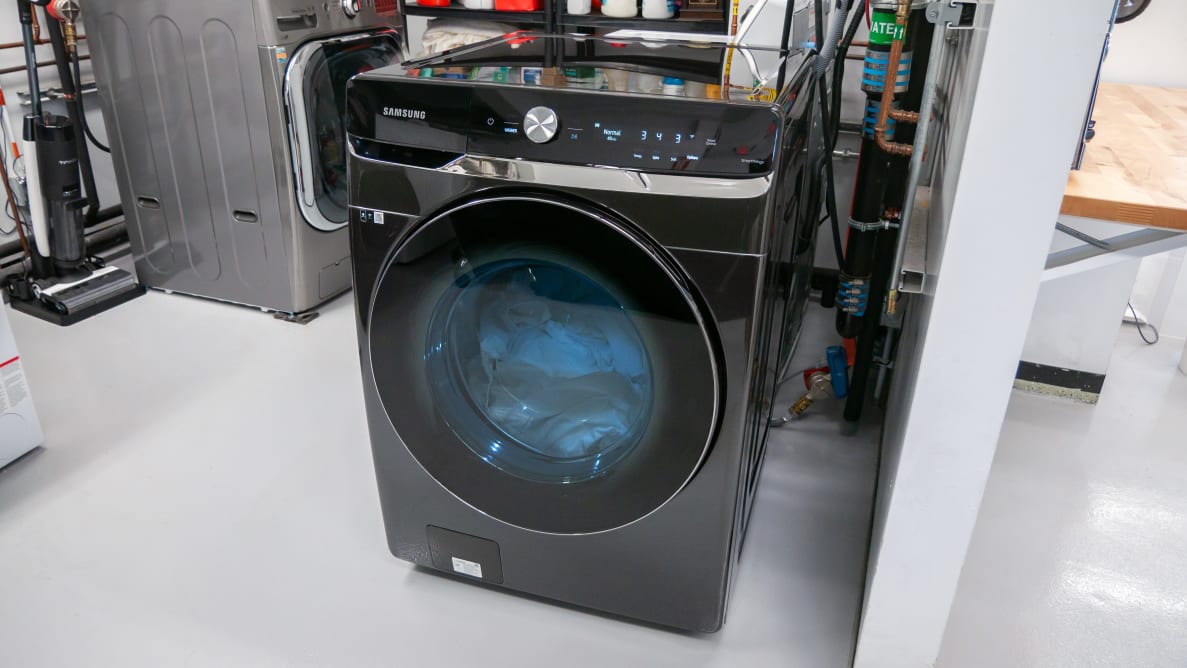This landscape-oriented, color photograph captures a Samsung side-loading washing machine centrally positioned in an indoor utility space, likely a laundry room. The washing machine, which is black and dark grey, features a silver dial centrally located on its top panel and a digital display screen to the right showing the numbers "3," "4," and "3." The round, transparent door on the machine's front reveals white clothing inside. The top left of the machine's panel prominently displays the white Samsung logo. The room’s utility nature is underscored by visible water piping behind the washer and a black vacuum cleaner located toward the back left near a white wall. Additionally, there is a glimpse of another machine, possibly a dryer, next to the Samsung washer. Utility shelves and a gray cabinet are partially visible, completing this detailed depiction of a functional, cluttered laundry space.